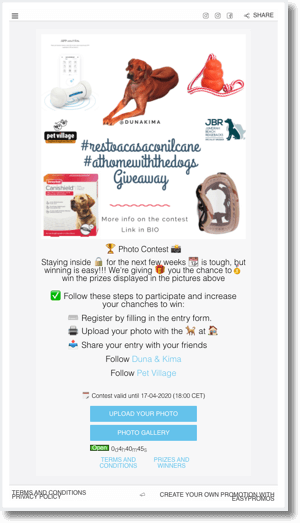A shadowy figure occupies the right side of the image, shrouded in darkness. The bottom left corner contains text that reads "Terms and Conditions, Privacy Policy," along with a logo that says "Create Your Own Promotion with Easy Promos." A subtle overlay text asks "How Are We Going to Use Them?" suggesting a possible gear-related promotion. On the left side of the image, there's a clear depiction of a sleek electronic device. In the foreground, a brown-furred dog chews on a colorful plastic toy shaped like various objects, amidst a vibrant scene labeled "Pet Village." The image also features a movie theater marquee displaying "JBR Movie Theater Showcase."

A delicious-looking meal catches the dog's attention as it looks at the food longingly. A text overlay mentions an exciting giveaway, but advises that more information on the contest can be found via the "link in bio." The image promotes a photo contest under the tagline "Staying Inside for the Next Few Weeks? Here's Your Chance to Win Prizes!" Participants are encouraged to register, upload their photos of their cats at home, and follow the account for more updates under the "Pet Village Contest" banner.